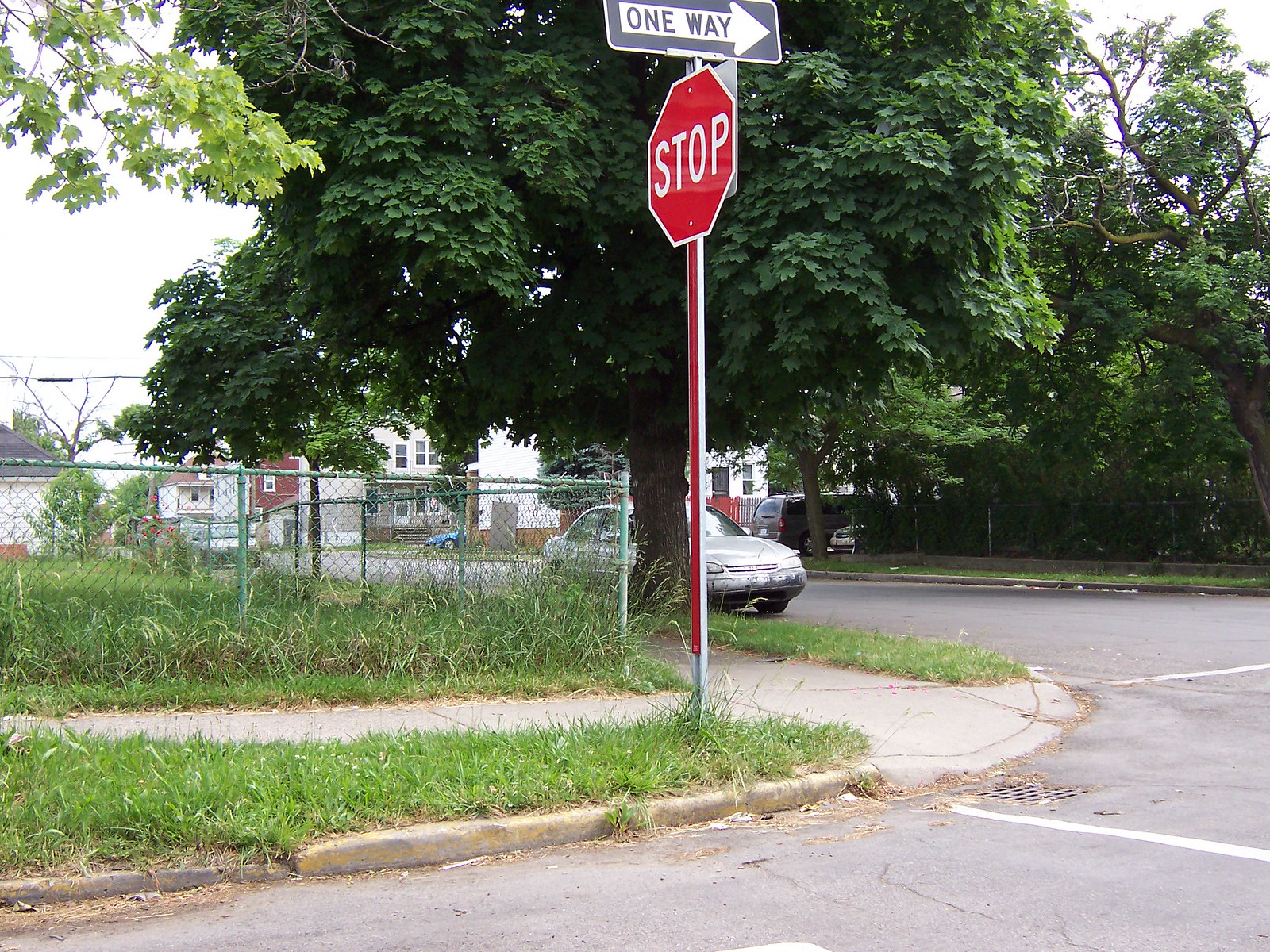In this real-life photograph taken at the corner of a suburban intersection on an overcast day, we see a detailed and bustling neighborhood scene. Dominating the image is a stop sign with its familiar red octagon shape and white capital letters that read "STOP." Above it, attached to the same pole, a rectangular one-way sign with a black background and a white arrow points to the right. 

The stop sign stands at the end of two intersecting sidewalks, surrounded by untrimmed, uneven grass that has grown quite long. The pavement of the street is faded blacktop, showing signs of age with visible cracks. White stop lines are painted on the asphalt marking the intersection.

In the middle of the scene, there is a large, leafy tree providing shade over a parked silver sedan. Multiple other cars are visible, lined up along the street and parked in driveways of the houses that line the road. The houses vary in appearance, but one noticeable house is partially visible behind a chain-link fence, which encloses a grassy area and extends along the sidewalk. 

The area has a mixture of greenery, including large trees with varying shades of green leaves. The sky overhead is light gray, indicative of a cloudy yet bright day, with hints of blue peeking through the cloud cover. The overall setting captures the serene yet vibrant essence of a typical suburban neighborhood.